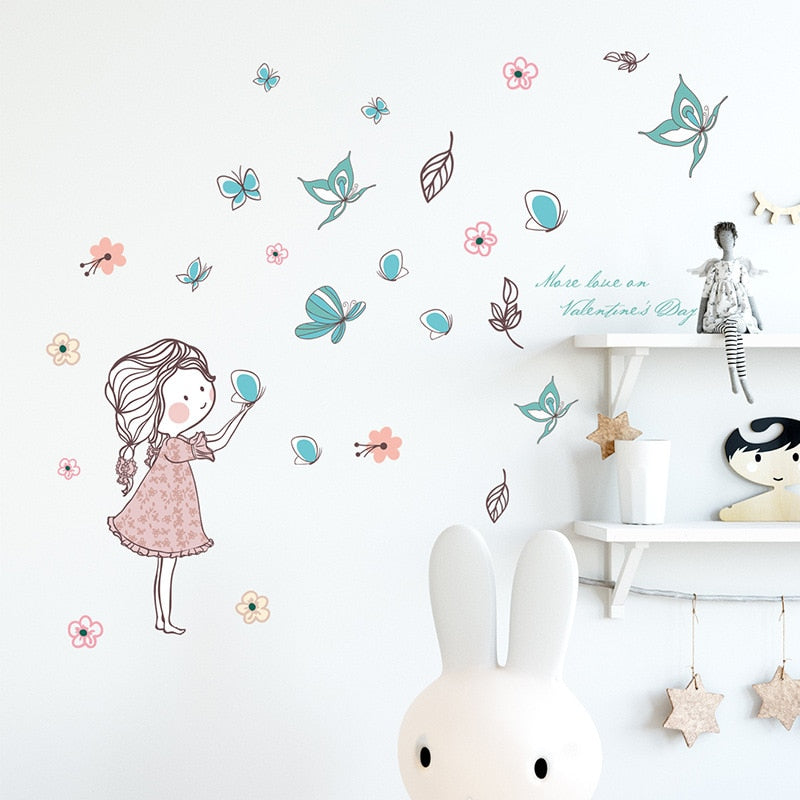This image showcases the detailed wall of a little girl's room, emphasizing an illustrated mural and charming decor. The mural, set against a white wall, features a cheerful little girl in a pink dress with her hair in a ponytail, delicately holding a blue butterfly amidst a flurry of butterflies in various colors, including blue, pink, orange, and yellow. Surrounding her are playful cartoon flowers and leaves, adding a whimsical touch to the scene.

On the right side, two white wall shelves stand out. The top shelf holds an angel-like doll dressed in a floral outfit with black and white striped leggings, its legs playfully dangling over the edge. The bottom shelf supports a tall white cup with a star attached to it and a little sculpted doll face ornament. Directly beneath this shelf, a string of star decorations hangs, cascading down the wall. At the bottom, a white plastic bunny head with black eyes peeks into the frame, adding a final touch of character to this enchanting room. The decor pieces harmonize with the mural, creating a space that radiates warmth and imagination.